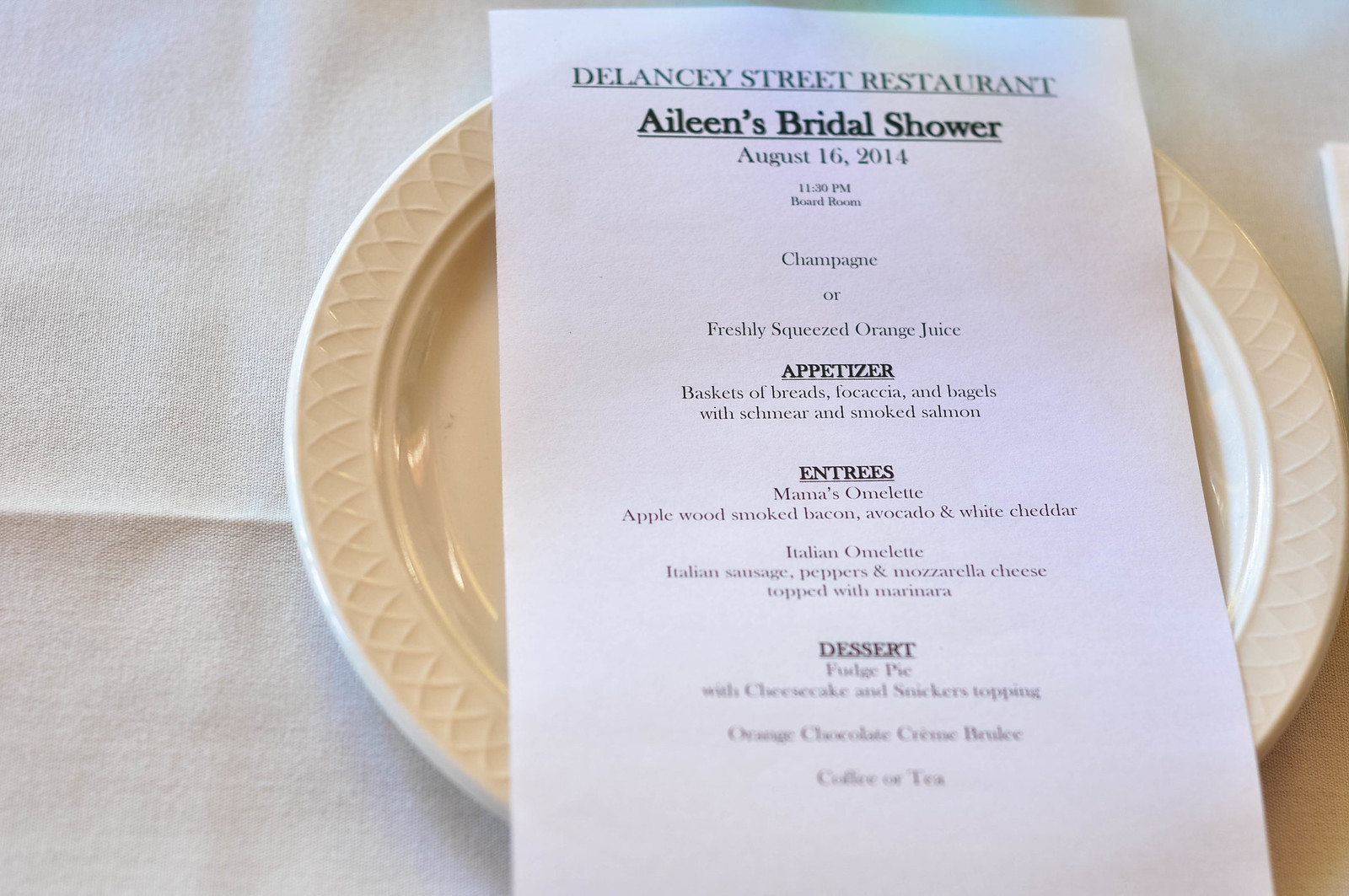This image is a top-down photograph taken at Eileen's Bridal Shower on August 16, 2014, held at the Delancey Street Restaurant. The scene is meticulously set with a white tablecloth hosting a neatly arranged white ceramic plate. Resting atop the plate is a standard-sized white paper menu printed in black text. The menu's headline reads "Delancey Street Restaurant," followed by "Eileen's Bridal Shower," both underlined and prominently displayed. Below this, the date "August 16, 2014" is noted. The menu offers a choice of Champagne or freshly squeezed orange juice to start. The appetizers include a variety of breads and focaccias with shmear and smoked salmon. The entrée options feature Mama's omelette with applewood smoked bacon, avocado, and white cheddar, and an Italian omelette with Italian sausage, peppers, mozzarella, and marinara sauce. Desserts listed are fudge pie with cheesecake and Snickers topping, and orange chocolate creme brulee, followed by an offer of coffee or tea. The well-lit photo, likely captured using a smartphone by a guest, showcases all these details clearly against its clean, monochromatic backdrop.